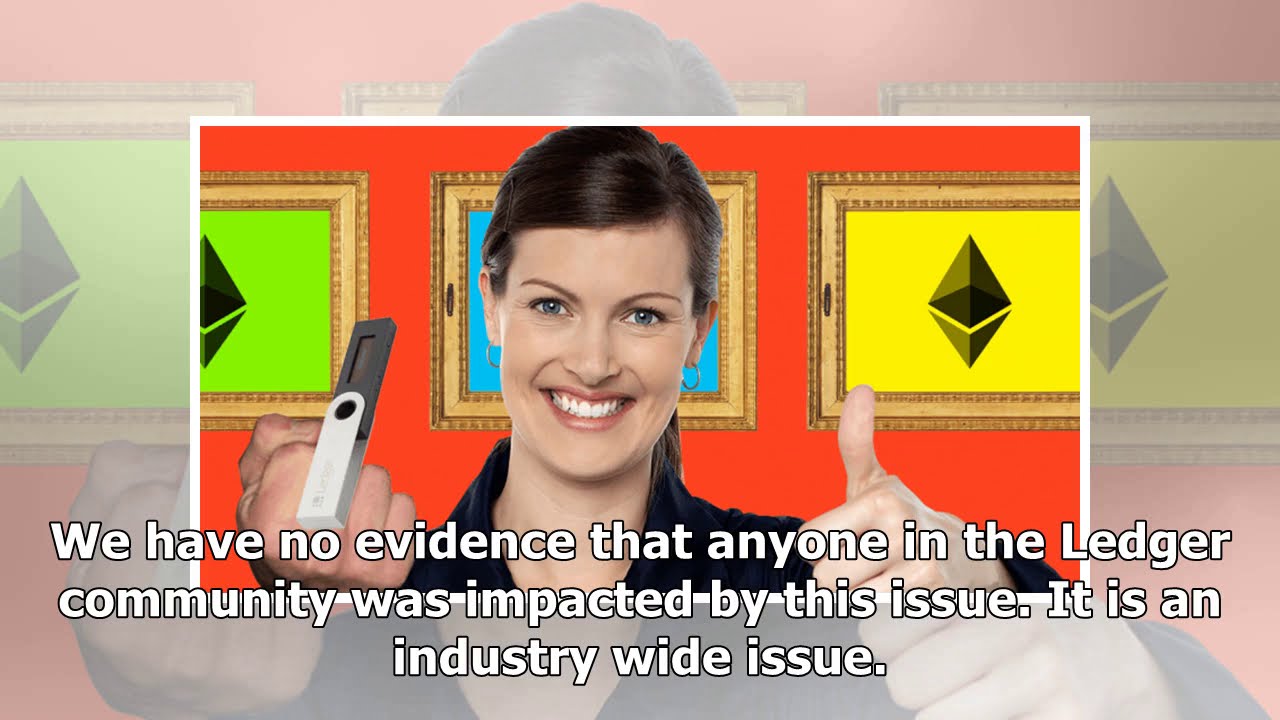The image showcases a smiling Caucasian woman, likely in her late twenties, with straight brown hair pulled back into a ponytail and adorned with small earrings. She has gray-blue eyes, pink lipstick, and is dressed in a navy or black shirt. Her left hand extends forward in a thumbs-up gesture, while her right hand seems to be giving a middle finger, though it is obscured by what appears to be a black and white USB drive.

The setting is an office-like environment with an orangish-red wall behind her. This wall features three framed pieces of artwork in vintage gold frames. The artwork includes a green background with a gray diamond on the left, a blue background with a gray diamond in the center, and a yellow background with a gray diamond on the right.

An overlay of white text on the image reads, "We have no evidence that anyone in the Ledger community will be impacted by this issue. It is an industry-wide issue." The background of the photo is a blown-up, faded version of the central image, giving it a surreal, possibly satirical quality.